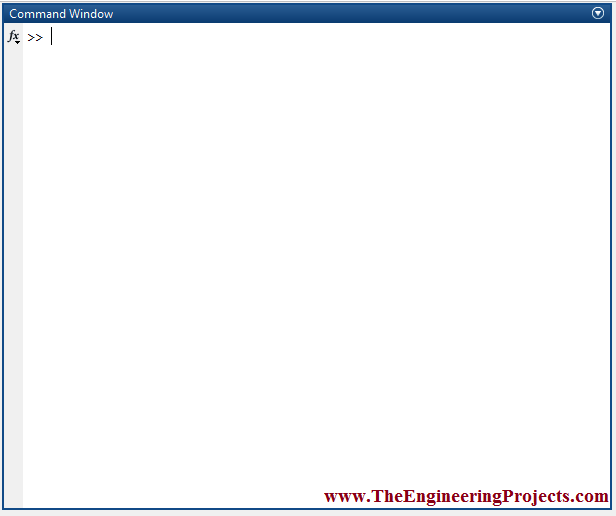**Caption:**

The image depicts a command window interface with a blue border running along the top. At the top of the window, it prominently displays the title "Command Window" alongside a distinct icon. Below this, the text "FX" is visible, followed by two greater-than symbols (">>"). A blinking cursor is present, ready for input. The left side of the window is framed by a light gray vertical border running from top to bottom. The majority of the window is an empty white space, devoid of any content, except for the bottom right corner where the URL "www.theengineeringprojects.com" is written in red text. The entire window is encased by a blue border along the top, bottom, left, and right edges, contrasting with the predominantly white interior space.